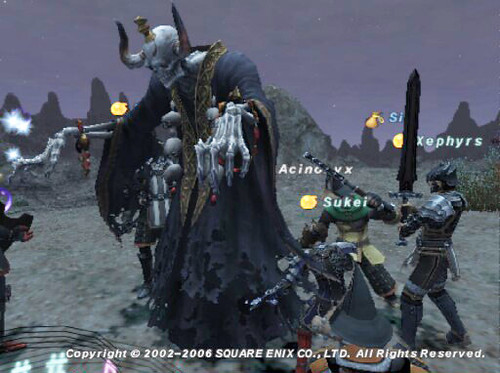This image is a screenshot from an early 2000s fantasy video game, as indicated by the copyright line at the bottom of the screen: "© 2002-2006 Square Enix Co., Ltd. All rights reserved." The scene depicts a dramatic battle set in a medieval, fantastical world. At the center, a towering skeleton figure draped in an intricately detailed black cloak with gold embroidery dominates the scene. The skeleton, adorned with horns on its head and various pieces of gold jewelry, stands ominously with large skeletal hands. The creature's eyes are fixed downward, appearing to be the primary boss or enemy that players need to defeat.

Surrounding the formidable skeleton are three knights, each uniquely armored and caught in the heat of battle. On the right side of the image, a knight in full armor brandishes an oversized sword above his head, poised to strike. To his immediate left, another knight, this time without a helmet, prepares for combat. Further to the left, a third figure, dressed in distinctive green and yellow armor, engages in the fight. The names "Suke," "Asino," "Onyx," and "Zephyrus" float above their heads, suggesting that this is a multiplayer game with different players controlling each knight.

The background sets a dark, moody atmosphere with a sky painted in shades of purple and blue and distant towering cliffs. The ground beneath these warriors is barren and gravelly, fitting the overall desolate landscape where this epic battle unfolds.